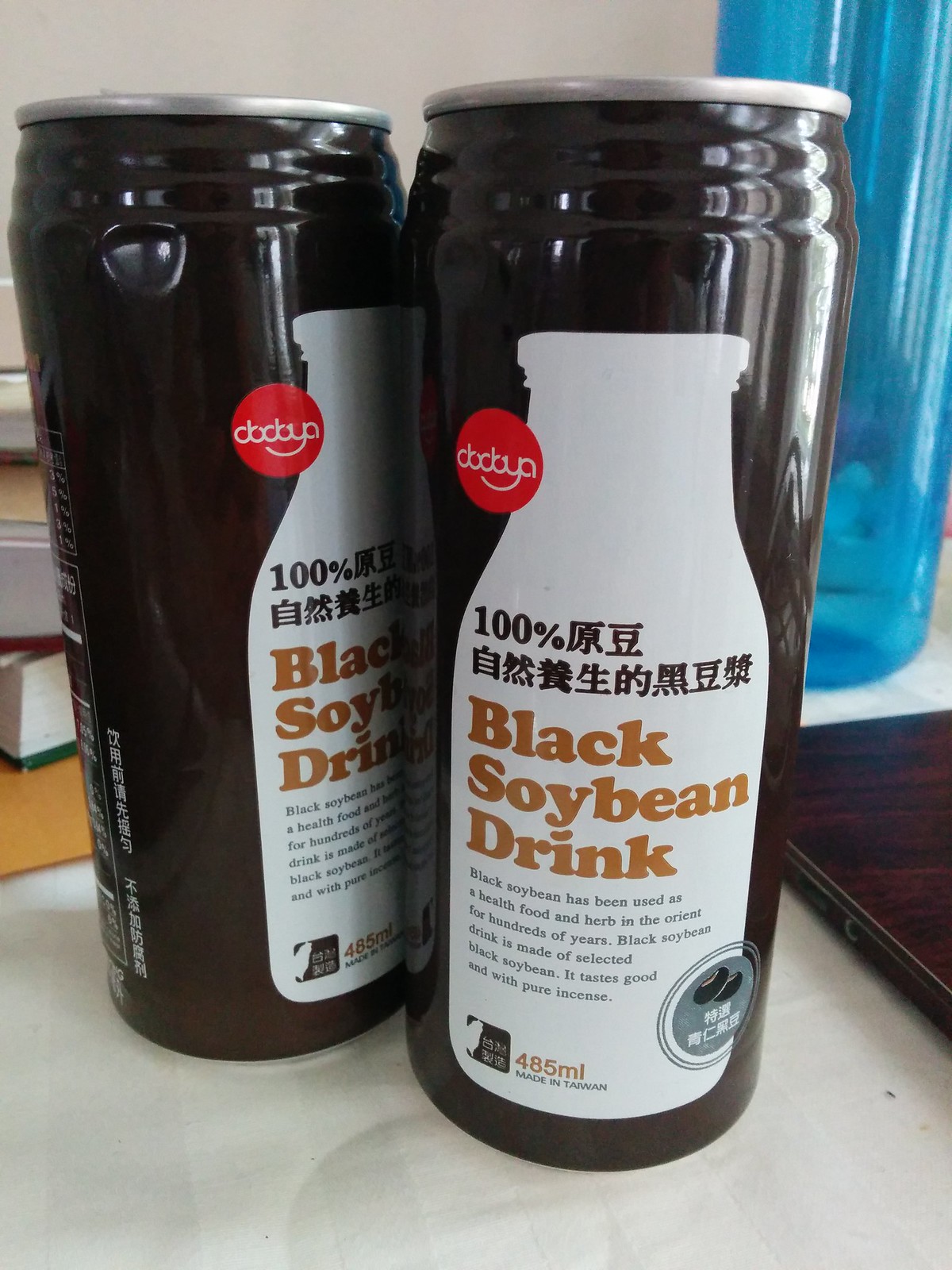This photograph features two aluminum cans with a dark chocolate-brown color. The cans have shiny aluminum tops and the label prominently displays "100% Black Soybean Drink" in English, with additional text in Chinese characters. Below the main label, there is a description in black text that reads, "Black soybeans have been used as a health food and herb in the Orient for hundreds of years. This black soybean drink is made of selected black soybeans, tastes good, and has a pure essence." Each can contains 485 milliliters of the beverage and indicates it is made in Taiwan. The cans are placed on what appears to be a countertop, desk, coffee table, or end table.